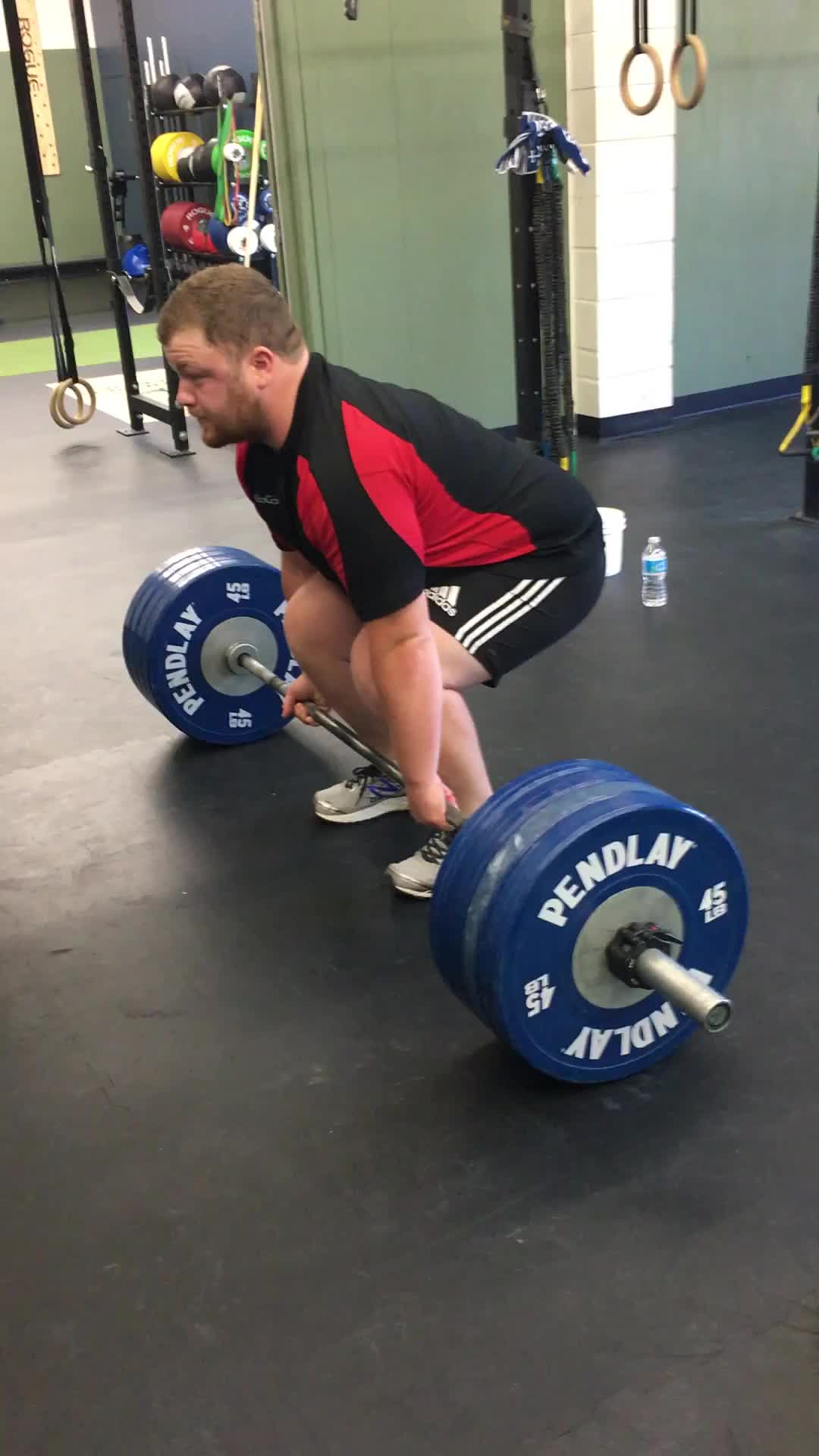This color photograph, taken in portrait format, captures a determined Caucasian man in his late 20s or early 30s preparing to lift a heavily loaded barbell in a gym setting. He is squatting down with one hand gripping the bar forward and the other hand back, about to perform a deadlift. He is dressed in black Adidas shorts with three white stripes on the side, a sporty red and black top, and sneakers. Sporting a close-cut beard and clean-cut hair, the man's expression conveys concentration and effort. The barbell, marked "Pendlay," is loaded with four to five 45-pound plates on each end. The gym's environment includes brick walls—some painted yellow and green—exercise rings hanging from the ceiling, and a variety of weights, kettlebells, and other gym equipment scattered around. A water bottle and a black rubber mat are visible on the floor, providing a safe and supportive surface for lifting.